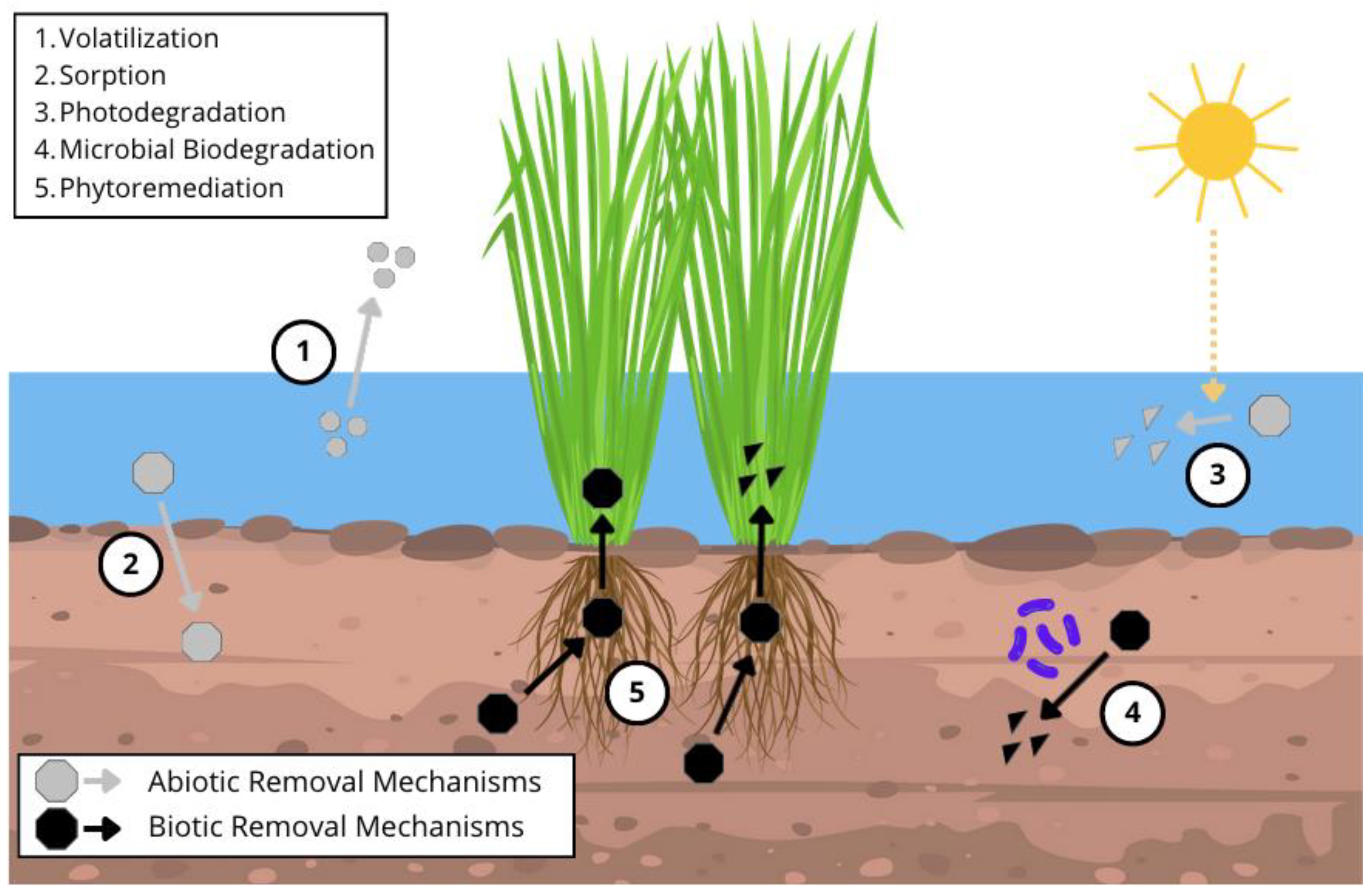This scientific diagram illustrates the mechanisms of abiotic and biotic removal processes. The central focus is on two tall green plants resembling tall grasses, partially submerged in water. Their brown roots extend downward into the soil beneath the water surface. A sun symbol is depicted above the water, indicating the influence of sunlight on the processes.

The diagram is annotated with five numbered circular labels (1 to 5), each connected by arrows to various parts of the scene, demonstrating distinct removal mechanisms. Label 1 represents volatilization, where contaminants transfer from water to the atmosphere. Label 2 denotes sorption, indicating the adherence of contaminants to soil particles or plant roots. Label 3 refers to photodegradation, the breakdown of contaminants through sunlight exposure. Label 4 signifies microbial biodegradation, the decomposition of contaminants by soil microorganisms. Lastly, Label 5 marks phytoremediation, where plants absorb, transform, and contain environmental pollutants.

Overall, the diagram effectively communicates the interplay between abiotic and biotic processes in removing contaminants from an aquatic environment.